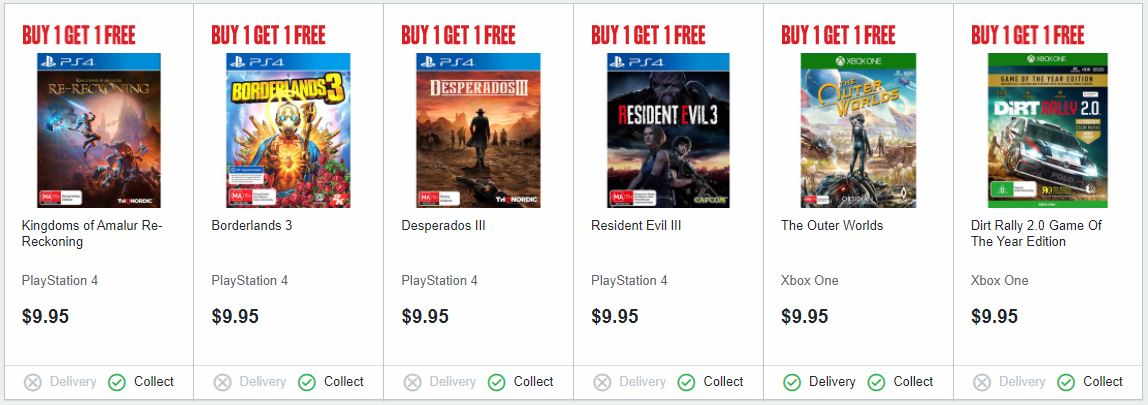This sales page for video games showcases a range of titles available for a special "Buy One, Get One Free" promotion. Displayed across the top of the page, this offer is advertised above each game's cover image. The lineup includes:

1. **Kingdoms of Amalur: Re-Reckoning (PS4) - $9.95**
   - The cover features a character battling a creature on a planet with a striking red and orange mountainous backdrop. Delivery is unavailable (marked by an "X"), but the game is available for collection (indicated by a checkmark).

2. **Borderlands 3 (PS4) - $9.95**
   - The cover image shows a masked figure. Like the other titles, delivery is not an option (marked by an "X"), though collection is available (checkmark).

3. **Desperados 3 (PS4) - $9.95**
   - This game cover depicts a Western setting with a central figure wearing a cowboy hat and several characters and a typical Western landscape in the background. Delivery is unavailable (marked by an "X") but is available for collection (checkmark).

4. **Resident Evil 3 (PS4) - $9.95**
   - The cover features two armed characters standing prominently. Again, delivery is not offered (marked by an "X"), but the game can be collected in-store (checkmark).

5. **The Outer Worlds (Xbox One) - $9.95**
   - The game cover shows a character wielding a weapon. Similar to the others, this title is not available for delivery (marked by an "X"), but it can be collected (checkmark).

6. **Dirt Rally 2.0: Game of the Year Edition (Xbox One) - $9.95**
   - The cover sports an image of a rally car. Delivery is not available for this game (marked by an "X"), but in-store collection is an option (checkmark).

Each title is priced at $9.95 and, due to the promotion, offers customers a chance to buy one game and get another one of equal or lesser value for free.